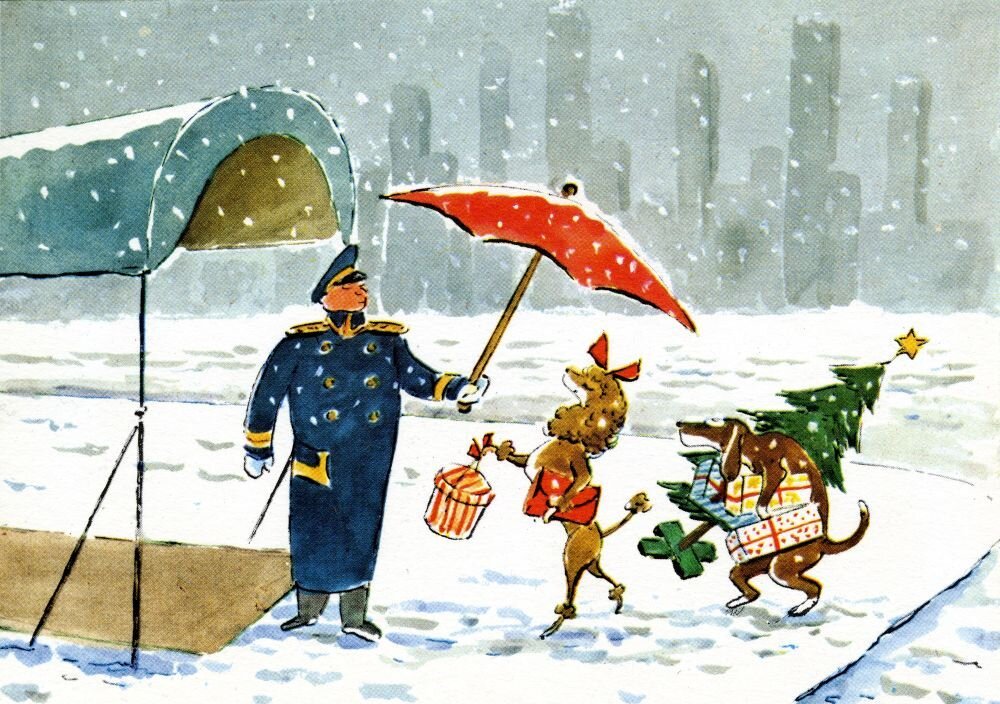The image is a whimsical, colorful illustration, reminiscent of a New Yorker magazine style from the 1940s. It captures a snowy winter day on the outskirts of a bustling city, likely New York, with tall buildings faintly visible in the background. In the foreground, a polished doorman dressed in a blue suit with gold buttons, golden shoulder pads, and white gloves stands beside a blue-gray awning. He is holding a large red umbrella, shielding an anthropomorphic poodle from the falling snow. The poodle, adorned with a red bow, is elegantly walking on her hind legs, carrying a red handbag and a red-and-white striped hat box. Behind her is a brown dog with white spots, struggling to balance a small Christmas tree topped with a yellow star and several Christmas packages—one wrapped in blue and white, another in yellow and white, and the last in red and white speckles. The dogs are making their way towards the covered entrance, seeking shelter from the snow-laden cityscape. The scene is festive and lively, evoking a sense of holiday cheer and the hustle and bustle of city life.